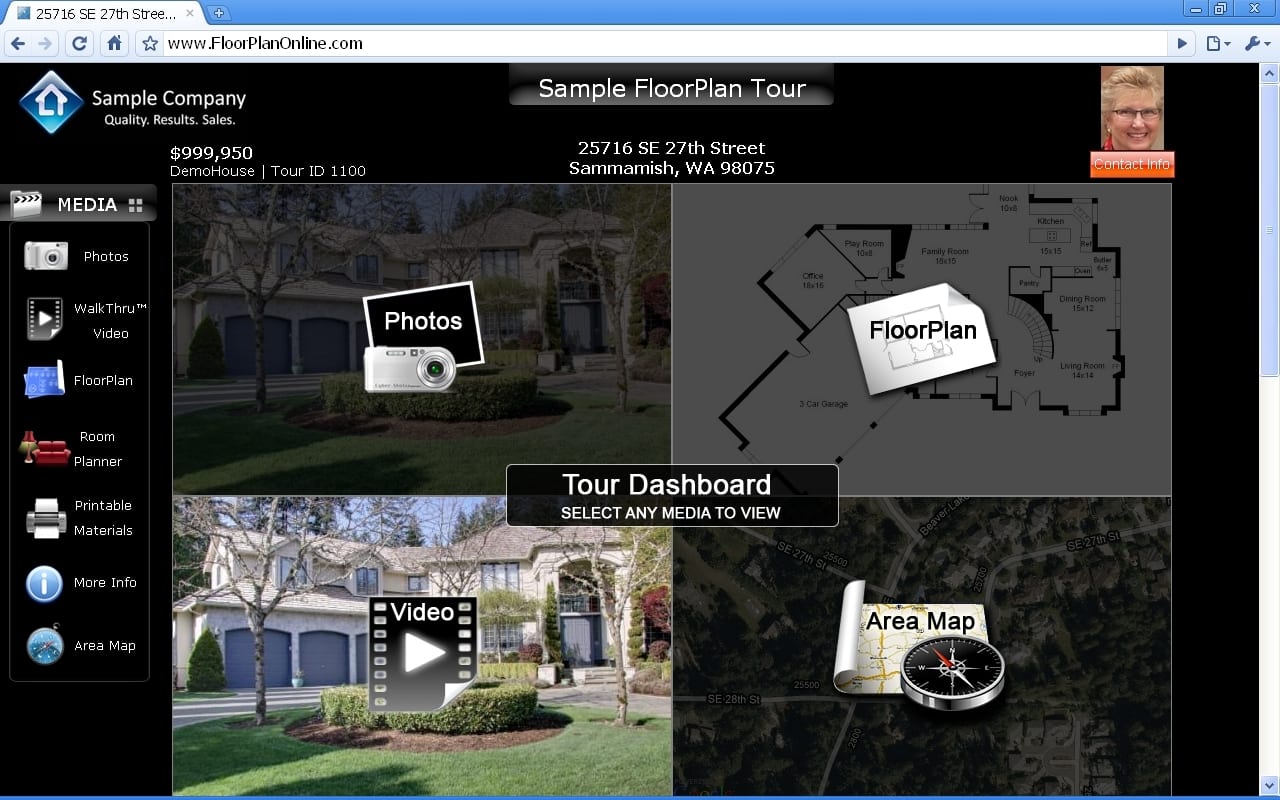This image showcases the website of a sample company with a specific focus on floor plans. In the upper left-hand corner, the folder's address is displayed, accompanied by a small icon of a blue square. Below this, a highlighted left arrow is visible, followed by a refresh icon, a home icon, and a star icon from left to right. 

Central to the image is a search bar beginning with "www.floorplanonline.com," immediately below which the text "Sample Company" is displayed. Adjacent to this on the left, an angled blue square icon featuring a house symbol is present, rendered in a two-tone fade effect. Beneath the company name, the slogan "Quality Results Sales" is printed.

Dominating the middle section is the text "Sample Floor Plan Tour" along with the address "25716 SE, 27th Street," followed by additional address information. On the right side of this section, there is a photograph of a blonde woman with short hair and glasses.

To the left of the photo, the menu options include "Media" (which is highlighted), "Photos," "Walkthrough Video," "Floor Plan," and "Room Planner." Further down, icons corresponding to these menu choices are displayed, along with additional categories. Four media thumbnails are shown, labeled as Photos, Floor Plan, Video, and Area Map.

Centered in the image, the term "Tour Dashboard" is prominently displayed.